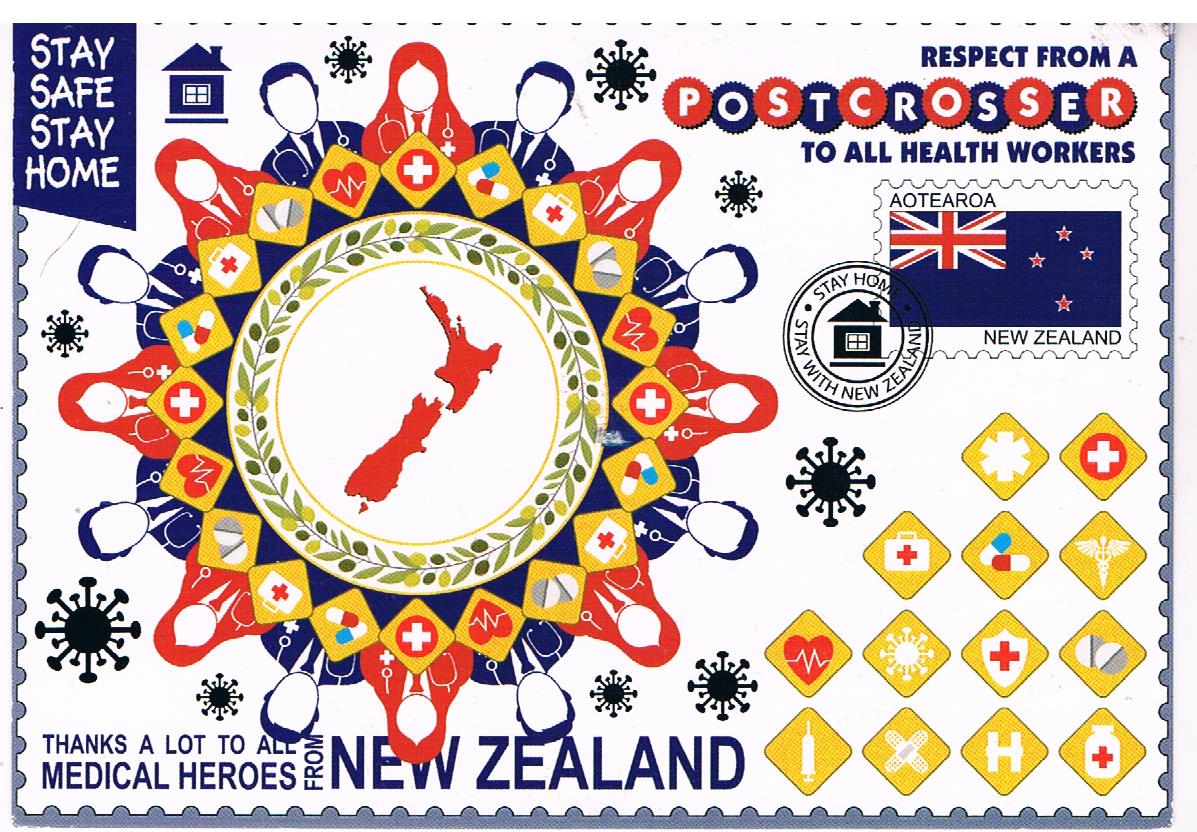This image resembles a postcard, featuring a detailed tribute to healthcare workers, likely created during the pandemic. Dominating the left side is an outline of New Zealand surrounded by a wreath of leaves and fruits. Surrounding this central image, silhouettes of healthcare workers—women in red and men in blue—all adorned with stethoscopes, symbolize medical professionals. Various small diamond icons depicting medical symbols such as a red cross, pill bottles, syringes, a heart, and first aid kits embellish the scene.

In the upper left corner, white letters on a blue rectangle instruct viewers to "Stay home, stay safe," while the upper right corner presents a message: "Respect from a post-crosser to all health workers," alongside a New Zealand stamp and flag. At the bottom, the text "Thanks a lot to all medical heroes from New Zealand" expresses gratitude. Black illustrations of bacteria float in the background, reinforcing the pandemic context and the encouragement to remain home. The image serves as a comprehensive and heartfelt salute to the dedication and bravery of healthcare providers.